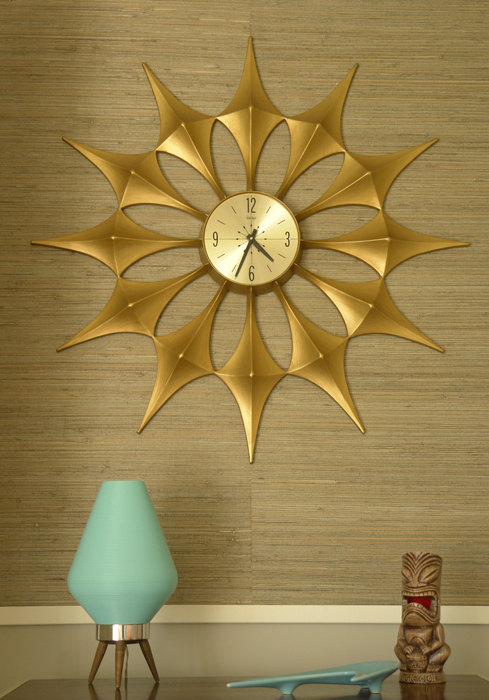The image features an intricately decorated wall with distinct details including a large, golden sunburst clock as the focal point. The clock, with a central gold face, displays the numbers 12, 3, 6, and 9 in black, alongside black hands indicating the time 4:34. This sunburst clock is characterized by spiky, diamond-shaped points resembling sun rays emanating from its center. The wall behind the clock features horizontally striped wallpaper in various shades of brown and beige, resembling bamboo.

Below the clock, a small, reflective wooden table hosts multiple decorative objects. To the left, there's a unique lamp piece with a turquoise vase-like structure atop a golden platform with tripod legs. Centrally positioned on the table is a crescent-shaped turquoise pottery piece, and to the right, a brown tiki mug adds an ancient, tribal aesthetic. The overall composition blends modern and tribal elements, set against a warm, textured backdrop.